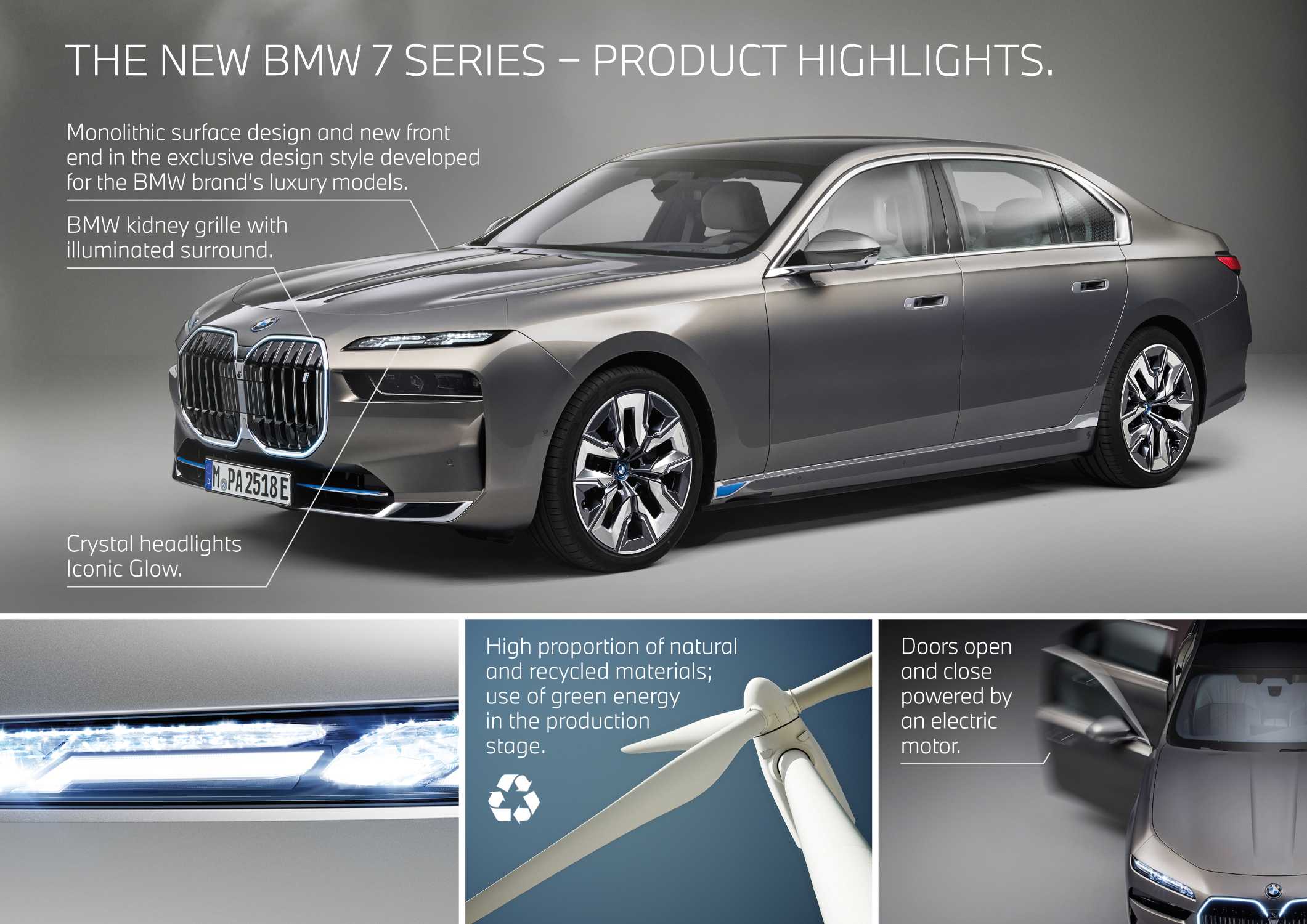The image showcases an advertisement for the new BMW 7 Series. At the top, in white lettering against a gray background, it reads "The New BMW 7 Series Product Highlights." The prominent feature of the ad is a sleek, silver-gray BMW car with bright silvery rims, and a license plate labeled PA2518E. The text highlights the car's "Monolithic Surface Design" and a "New Front End in the Exclusive Design Style Developed for BMW Brand's Luxury Models." It also emphasizes the "BMW Kidney Grille with Illuminated Surround" and "Crystal Headlights with Iconic Glow," showcasing the vehicle’s distinctive thin headlights.

Below the main image of the car, there are three smaller images. The first is a close-up of the headlights, highlighting the intricate design. The second image has a blue background and features a wind turbine and recycling symbol, with accompanying text that states, "High Proportion of Natural and Recycled Materials. Use of Green Energy in the Production Stage." The last image shows the car’s doors opening automatically, with text indicating, "Doors Open and Close Powered by an Electric Motor." Together, these elements provide a comprehensive overview of the luxury, innovative design, and environmentally conscious manufacturing of the BMW 7 Series.